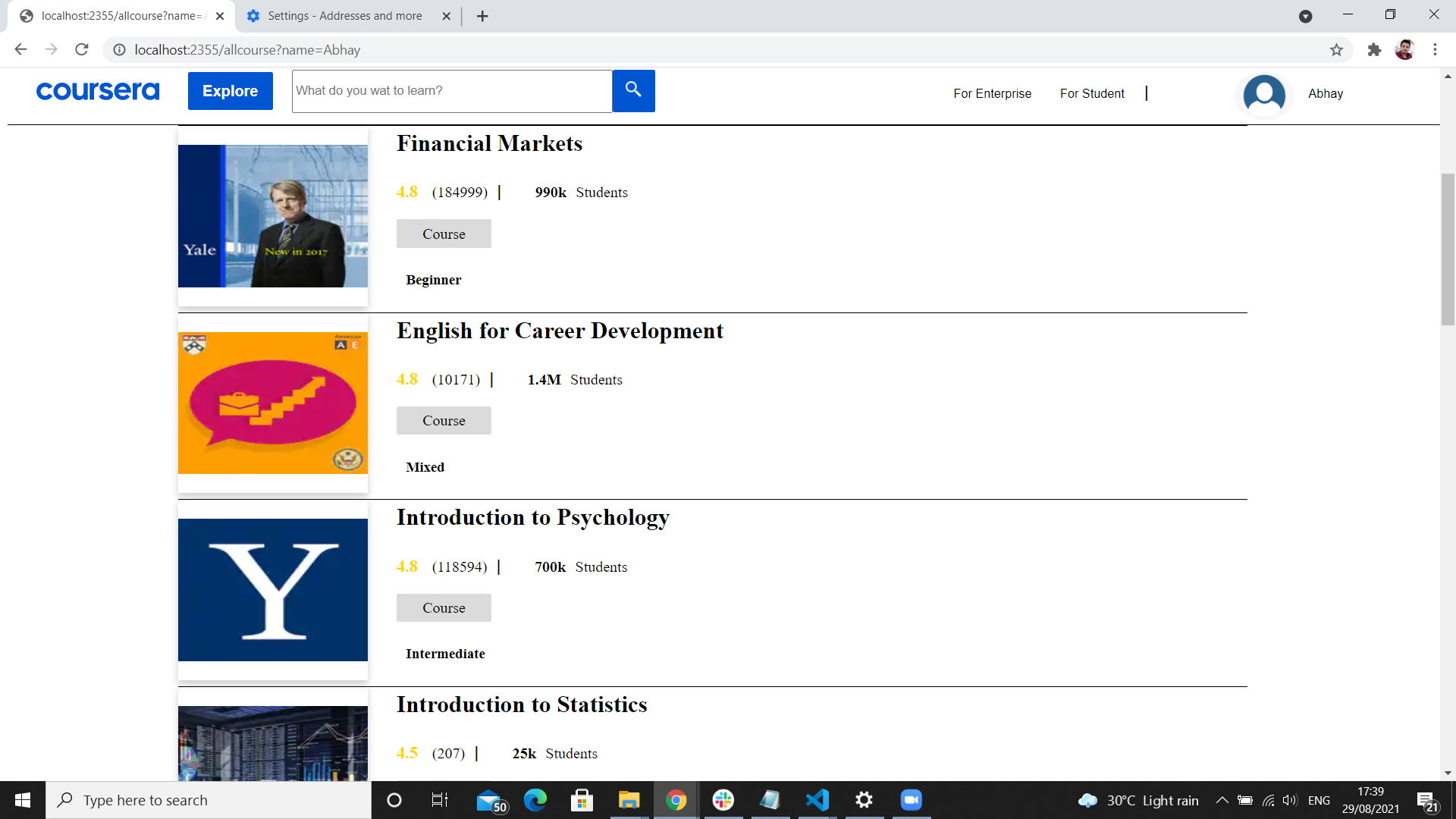The image showcases an open internet browser window with two visible tabs. The selected tab displays the Coursera website, featuring a variety of courses. Notable courses include: 

- **Financial Markets**: Rated 4.8 stars from approximately 184,999 reviews and has about 990,000 enrolled students.
- **English for Career Development**: Rated 4.8 stars with around 10,171 reviews and about 1.4 million enrolled students.
- **Introduction to Psychology**: Rated 4.8 stars based on 118,594 reviews and has roughly 700,000 enrolled students.
- **Introduction to Statistics**: Rated 4.5 stars with 207 reviews and approximately 25,000 students enrolled.

In the upper right corner, the user, identified as "Abhay," appears logged in. The browser interface indicates it is running on a Windows desktop, evidenced by the Windows logo in the lower left corner. The page primarily highlights the different courses Abhay is browsing on Coursera.